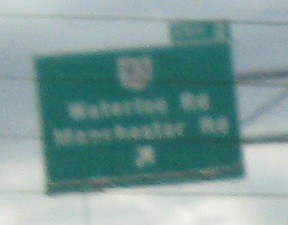A highly blurred image packed with various elements spanning from left to right. On the left side, there's a shield-like figure, under which some text can be faintly discerned, possibly stating "something row." Below that text, there's additional wording, also indiscernible, possibly echoing the previous line. An arrow pointing upwards is visible near the bottom. Dominating the top section, a green sign stands out, which seems to form the border of the image, accented by a blue hue at its upper edge. The lower portion of the image transitions to a predominantly gray tone.